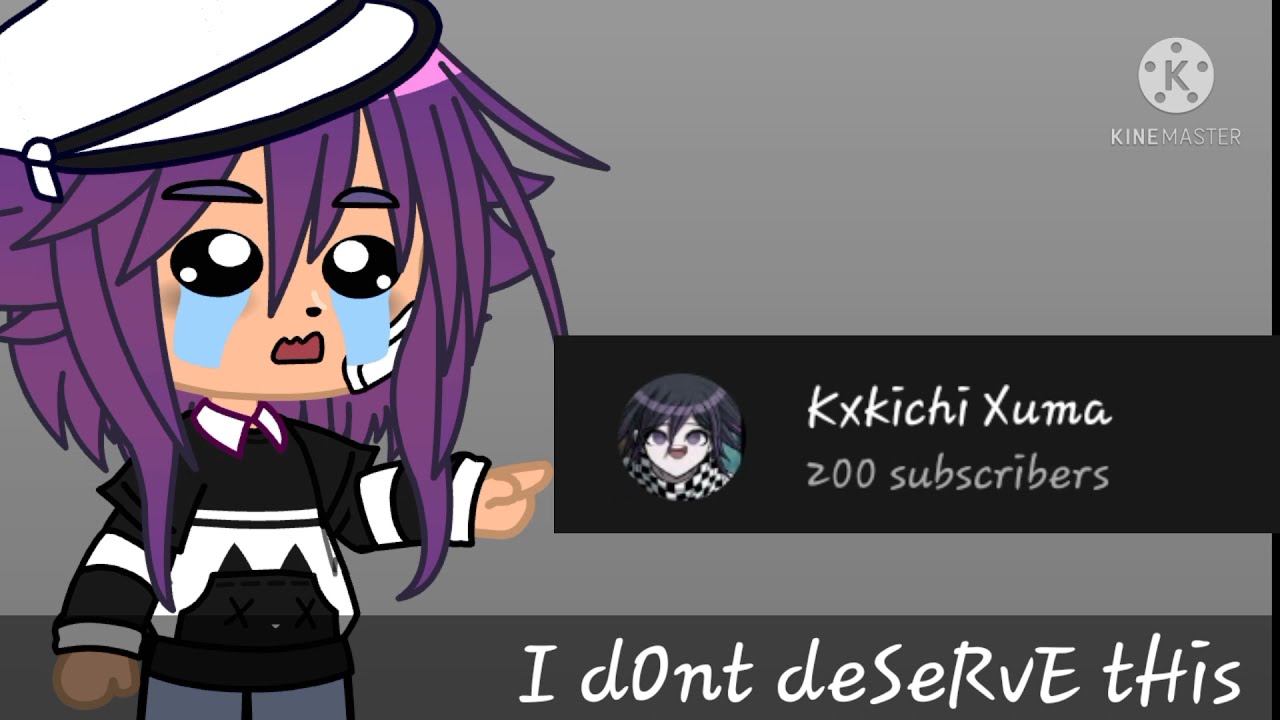The digital image features a character with long, jaggedy purple hair cascading just below the shoulders in some places and trimmed to shoulder length at the back. The character has prominent black eyes with two white circles within each eye, and appears to be crying, indicated by blue streaks under the eyes. Wearing a white hat with a black-trimmed brim, the character dons a black shirt featuring a white, Charlie Brown-esque jagged pattern along with a pocket that has black X marks. The shirt is layered over a long-sleeve black and white striped shirt. The character points to some text that reads "KXKICHI Exuma" along with "200 subscribers" below it, accompanied by an avatar of a person with black hair and a checkered shirt. The top right corner of the image bears a circular emblem with a 'K' inside, labeled "KineMaster." At the bottom, a white-font caption reads, "I don't deserve this." The entire scene is set against a gray background and has a distinct cartoonish style, reminiscent of Japanese animation.